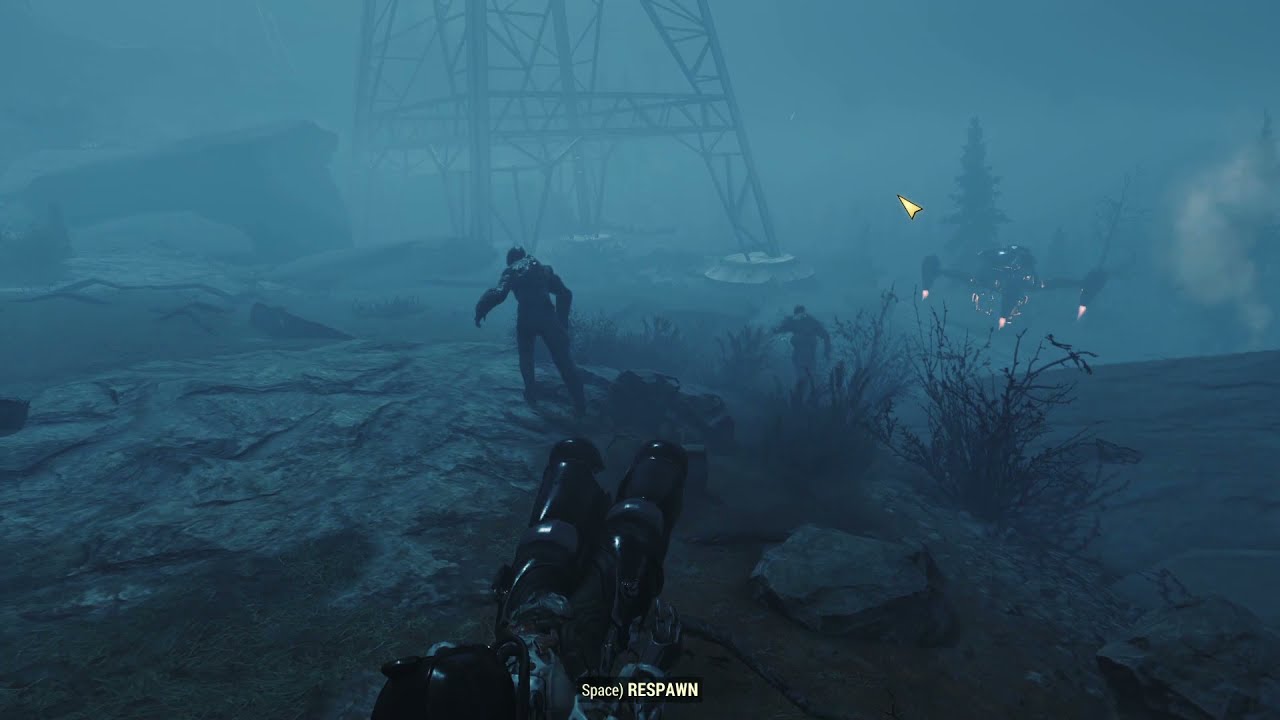In this detailed screenshot from a video game, we see an outdoor scene set on a hazy, dark night. The ground is composed of rocky, stone-like terrain with some sparse weeds scattered around. The overall color palette is tinted in various shades of blue, gray, black, white, and yellow, lending a cold and foreboding atmosphere to the scene. 

At the bottom of the screen, the text "space respawn" is visible, indicating that the player has died and needs to press the space key to respawn. This suggests the game is likely a third-person or first-person action game. 

Central to the image is a giant, metal tower rising prominently against the foggy backdrop. Off to the right-hand side of the screen, there is an aircraft or spaceship hovering near some smoky clouds, and nearby, what appears to be a tree-like structure. Above the spaceship, a mouse pointer is visible, indicating interaction with the game's interface.

In the foreground, two humanoid figures are walking away from what seems to be the player's perspective, which shows a first-person view of holding a gun. These figures are depicted as dark, monster-like creatures, one of whom is wearing a black suit with a helmet. Another person in the distance is also geared up, holding a weapon and seemingly wearing a helmet.

The overall impression is of a post-apocalyptic or sci-fi setting, rich in atmospheric tension and engaging details.